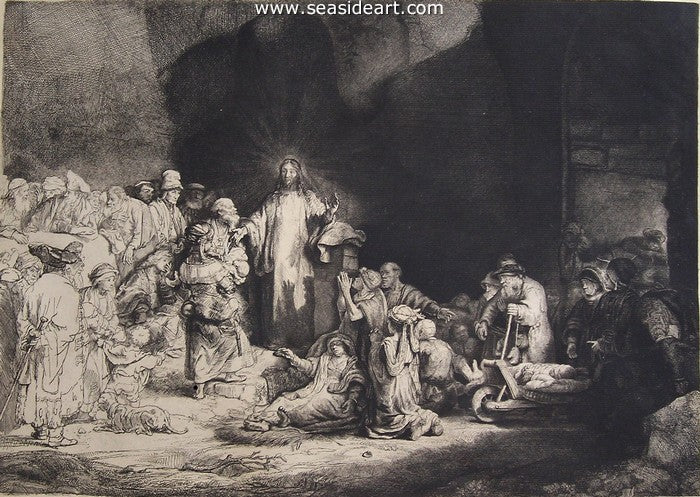In this detailed sepia-toned image, which bears the web address www.seasideart.com at the top, a figure resembling Jesus Christ stands central, garbed in a long, white robe with long dark hair. Rays of light radiate from behind his head, like a glowing halo, illuminating the scene. The artwork, possibly a pencil or graphite sketch, shows a gathering of people around him. These individuals appear to be a mix of the poor, sick, and those in need of assistance. Some are on their knees praying, while others stand or lie on the ground, exhibiting signs of illness or injury. Notably, there is a woman ascending steps toward him and an old man with a cane. The setting suggests an ancient, dim interior, perhaps a cave or stone structure, with shadows that accentuate the spiritual and somber atmosphere. In an old-fashioned stroller, a baby can be seen, alongside a dog on a leash. The floor is dirt-covered, with tree branches and rocks scattered about, further adding to the rustic and historical feel of the scene.